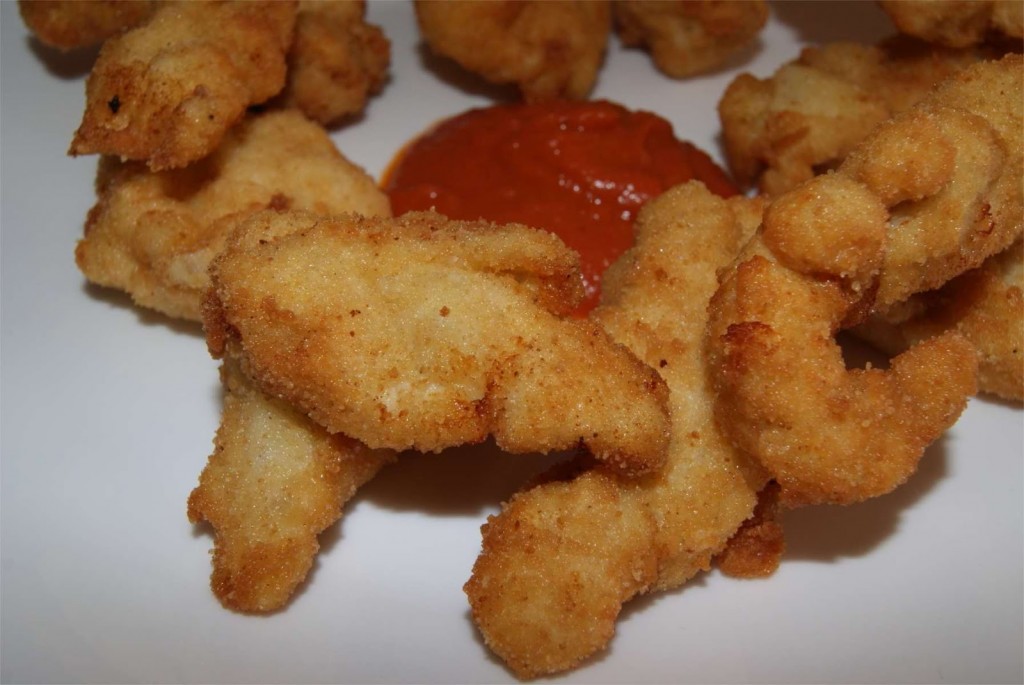This image showcases a close-up of a plate of lightly breaded chicken nuggets arranged in a circular pattern on a plain white plate. The golden-brown nuggets, approximately 10 to 12 in number, are stacked on top of one another, forming a ring around a central dollop of red sauce, likely ketchup. The nuggets, each roughly two inches long, appear crispy and well-cooked. The overall composition emphasizes the crispy, golden-brown texture of the chicken nuggets against the stark white plate, with the red sauce providing a contrasting focal point in the center. There are no other elements in the image, and the background details suggest a simple, homey setting, potentially someone’s kitchen.